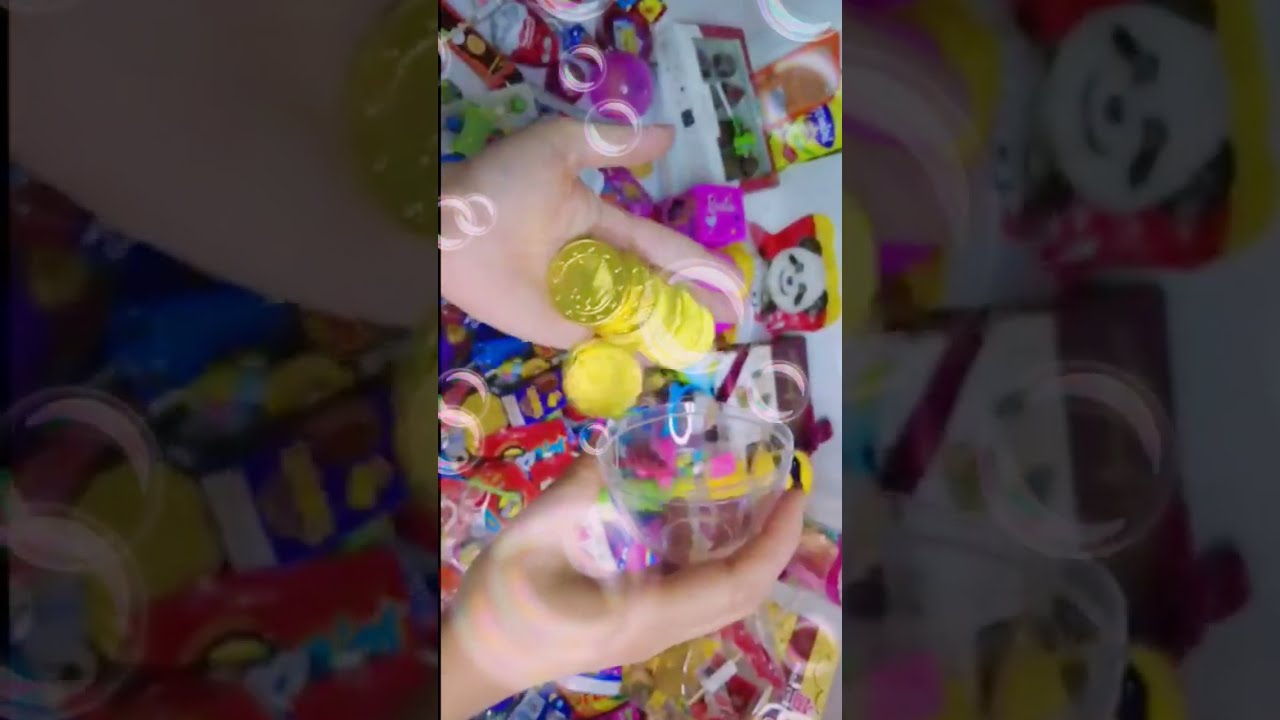The central image captures a pair of young, Caucasian hands holding an assortment of vibrant candy coins, predominantly gold but featuring colors like pink, green, blue, and yellow, possibly within a bag. This central portion is flanked by darker, identical segments from the middle picture. Surrounding this focal point is a colorful and chaotic array of party decorations, small toys, and vibrant balloons scattered across a tablecloth. Among these decorations, a purple box labeled "Barbie" and images of panda bears are visible. The image, possibly low-resolution, exudes a festive atmosphere, albeit slightly fuzzy, evoking a child’s birthday party immersed in joyful disarray.